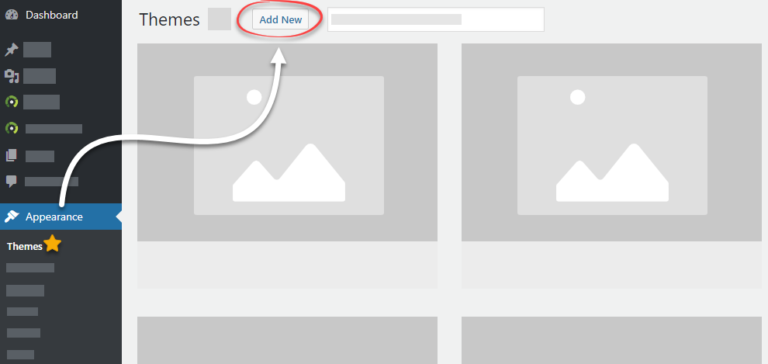The image appears to be a screenshot of a web interface related to theme management. At the top of the interface, there's a header labeled "Themes". To the right side of this header is a blue button with a gray outline that says "Add New". A red circle surrounds this button, drawing attention to it, and a white arrow points to it from the left, originating from a section that has a black background. 

Within this black section, there is a blue bar with the word "Appearance" written in white text, along with a small brush icon beside it. Below the "Themes" header, there are several placeholder images that depict a simple mountain and a sun illustration, arranged in two rows. 

At the top of the interface, positioned to the left, is a search bar. The left side of the image shows a black navigation area labeled "Dashboard" at the top. Below this, there are multiple icons including a pin, a green gear, a camera, a musical note, and a speech bubble. Under the "Appearance" section within the navigation area, "Themes" is displayed in white text alongside a gold star.